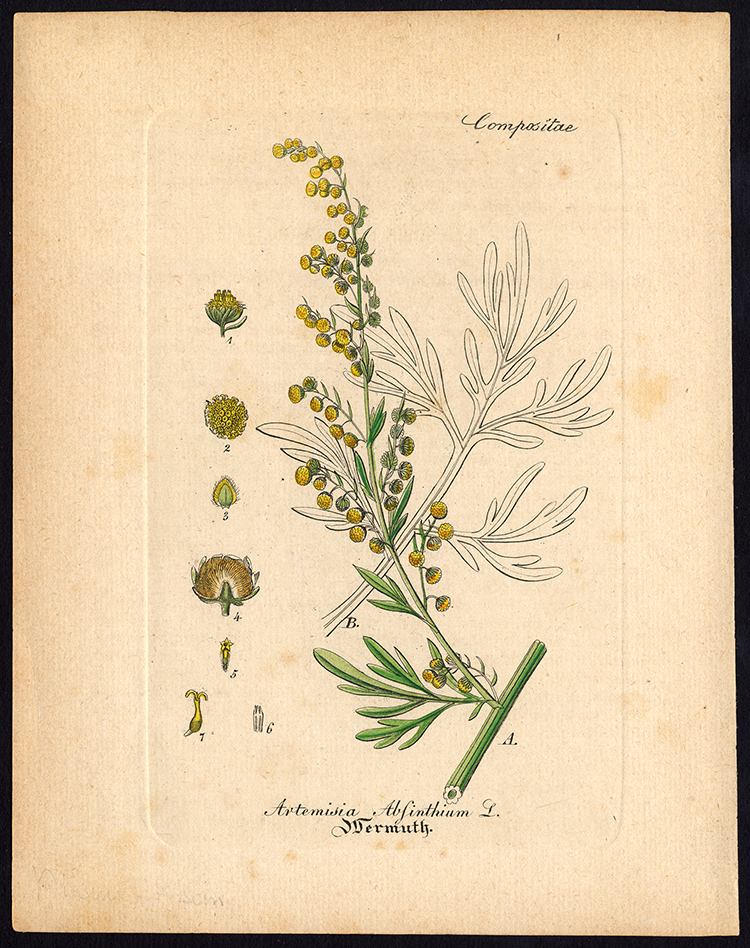The image is an antique-looking watercolor illustration of a plant, framed by a thin black border. The paper is aged, yellowed, and shows signs of wear with yellow spots. At the center of the image is a detailed depiction of a plant characterized by a long green stem with yellow flowers. There is also a small black-and-white sketch of the same stem intersecting the colored illustration, labeled with a 'B,' whereas the colored stem is labeled with an 'A'. To the left of the main plant illustration, seven smaller, intricately drawn sections of the plant are displayed, showing different views and life stages of the flowers, each labeled from 1 to 7. In the top right corner of the image, the word “composite” is elegantly written in cursive. At the very bottom of the illustration, the name of the plant, written in Latin, is partly discernable as "Artemisia althinium L fermentally."